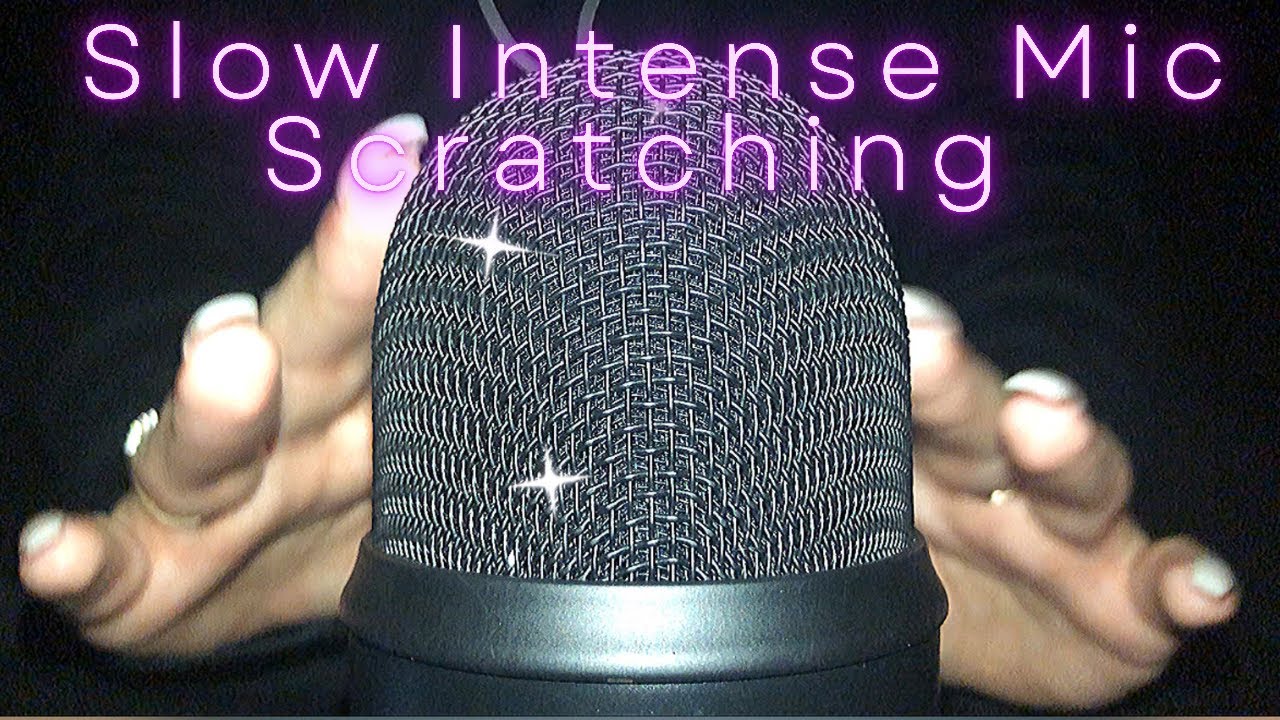A screenshot from an ASMR video features the text "Slow Intense Mic Scratching." The image showcases a close-up view of a microphone with two hands positioned behind it, their fingertips barely grazing the mic. The hands, belonging to a woman with long fingernails, suggest an upcoming ASMR session where she will meticulously and slowly move her fingernails down and around the microphone. This video epitomizes ASMR content, focusing on creating very quiet, soothing noises that require attentive listening. In this instance, the physical interaction with the microphone, characterized by delicate and intentionally slow scratching sounds, aims to provide a deeply relaxing auditory experience for ASMR enthusiasts.